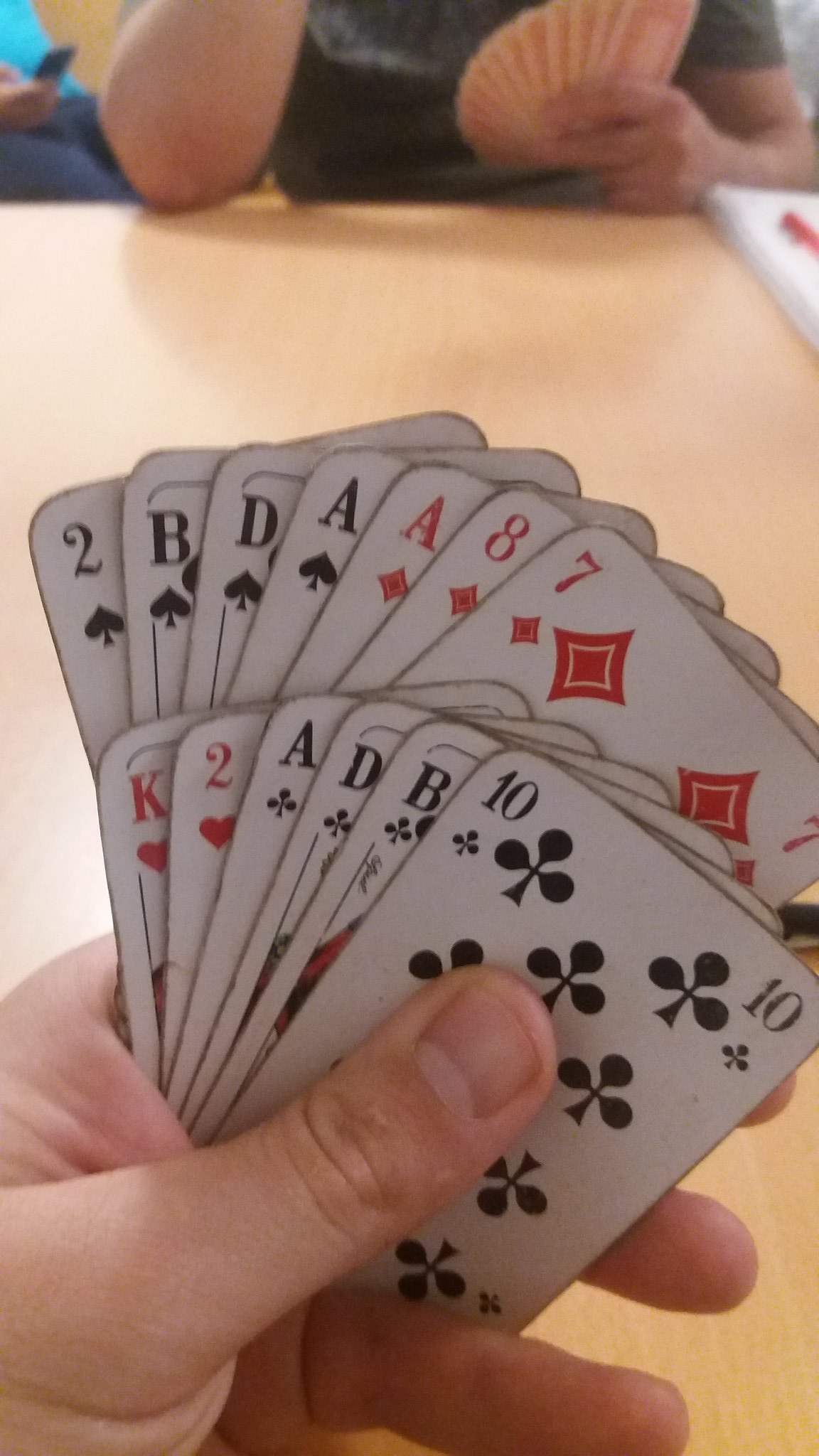In this image, a person is holding a set of cards in their left hand, arranged in two neat rows. The card arrangement includes, from left to right in the top row: a black '2', a black 'B', a black 'D', a black 'A', a red 'A', a red '8', and a red '7'. The second row at the bottom features a red king, a red '2', a black 'A', another black 'D', a black 'B', and a black '10'. The image isn't of the highest quality, but it is sufficiently clear to make out these details. 

In the background, at the end of the table, another person is also holding a bunch of cards, fanned out in their hands. On the upper right-hand corner of the table, there is a notebook and a pen, indicating that note-taking or scorekeeping might be involved. Another individual can be seen sitting in the upper left-hand corner of the image, seemingly uninterested in the card activity. The setting appears casual, contributing to the overall relaxed atmosphere depicted.